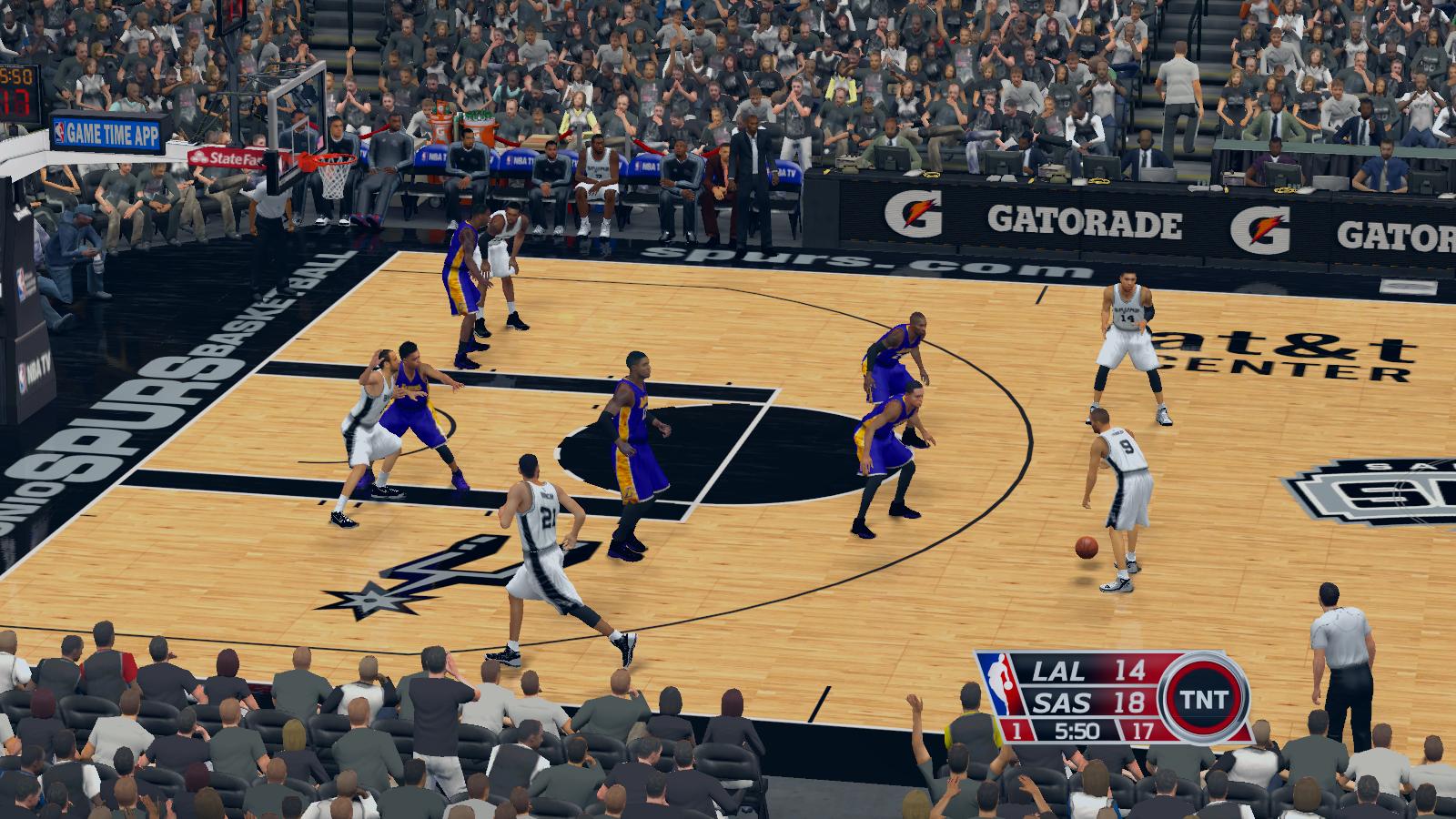This image is a detailed screenshot from a modern video game, showcasing a virtual basketball game set in the AT&T Center. The high-quality graphics allow for clear identification of the players, featuring notable San Antonio Spurs members: Tony Parker with the ball, Tim Duncan, and Manu Ginobili on the court. The scoreboard in the bottom right corner displays the NBA logo with the number "1," alongside the scores "L.A.L. 14" and "S.A.S. 18," with 5:50 remaining on the game clock and 17 seconds on the shot clock. The circular TNT logo, black and red, is also visible. 

The animated crowd in the background is dressed in a variety of outfits, predominantly in shades of brown, green, white, and black shirts with similar colored pants. Fans sporting white and black jerseys represent the Spurs, while others in purple and yellow jerseys support the Lakers. The AT&T Center logo is discernible in the upper right corner, while "Spurs.com" is prominently displayed along the sideline. The phrase "Spurs Basketball" is seen underneath the hoop, and the recognizable silver and black Spurs logo is situated on the left side of the court.